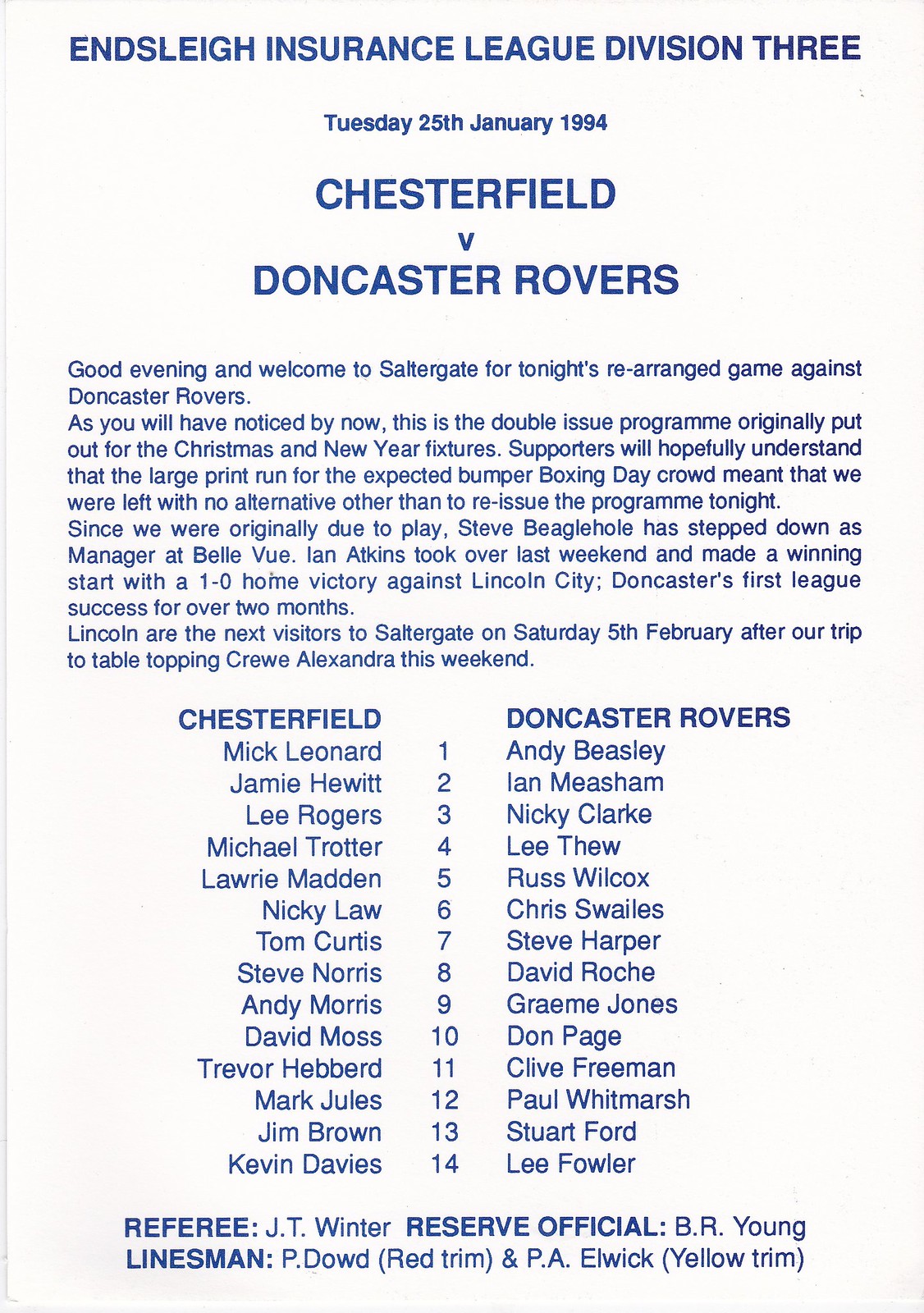This image depicts a page from the official game day program of the Ensleague Insurance League Division 3 match between Chesterfield and Doncaster Rovers, initially printed for the Christmas and New Year's fixtures but reissued for the January 25, 1994, game due to a large print run for the Bumper Boxing Day crowd. The match is held at Saltergate. The program opens with a welcome message noting that since the game was originally scheduled, Steve Beaglehole has stepped down as manager at Doncaster's Belle Vue, succeeded by Ian Atkins, who secured a 1-0 home victory against Lincoln City this past weekend—Doncaster's first league win in over two months. The next game at Saltergate will be against Lincoln on February 5, following Chesterfield's visit to table-topping Crewe Alexandra. The page also features the team rosters, listed vertically, for both Chesterfield and Doncaster Rovers, with columns dedicated to each. At the bottom, it lists the match officials: Referee JT Winter, Reserve Official BR Young, and Linesmen P. Dowd (Red Trim) and P.A. Eldwick (Yellow Trim).